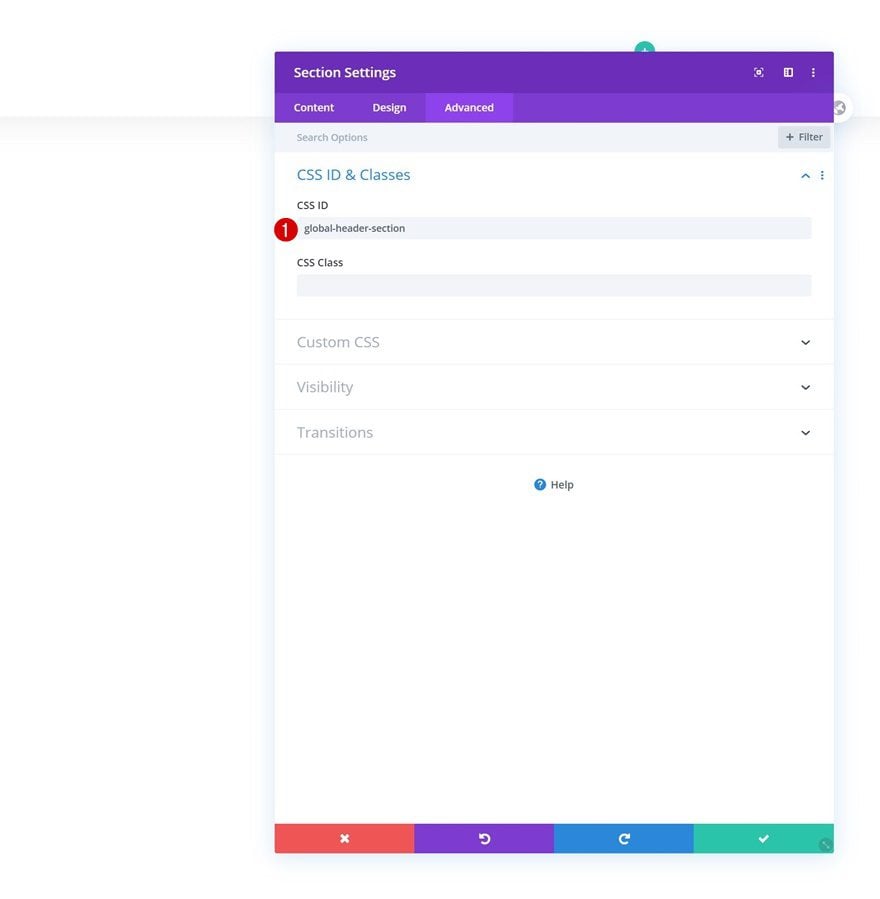The image is a screenshot of a software interface, possibly from a web design or development tool.

At the top of the screenshot is a bright purple bar with white text stating "Section Settings." Below this bar is another bright purple bar containing three buttons. From left to right, these buttons are labeled "Content," "Design," and "Advanced," with the "Advanced" button being highlighted.

Underneath these purple bars is a gray bar labeled "Search Options," featuring a 'Filter' button with a plus sign on the far right. The central area of the interface displays a prominent white box that contains text. At the top left of this white box, the text reads "CSS ID and Classes," followed by sections for "CSS ID" and "CSS Class." Next to the "CSS ID" section, there is a red circle with the number one inside and the text "Global Header Section." Under the "CSS Class" text, there is a gray bar for input.

Further down, three smaller white boxes are labeled "Custom CSS," "Visibility," and "Transitions." Directly beneath these sections is a small blue circle with a white question mark inside, signifying a 'Help' option. 

The bottom section contains a series of colored icons arranged in a horizontal bar. The first icon is a red box with a white 'X' symbol, indicating a delete or close function. The second icon is a purple box with an undo symbol (a white curling arrow pointing to the left). The third icon is a blue box featuring a redo symbol (a white curling arrow pointing to the right). The final icon on the right is a green box with a white checkmark, likely used for saving or confirming changes.